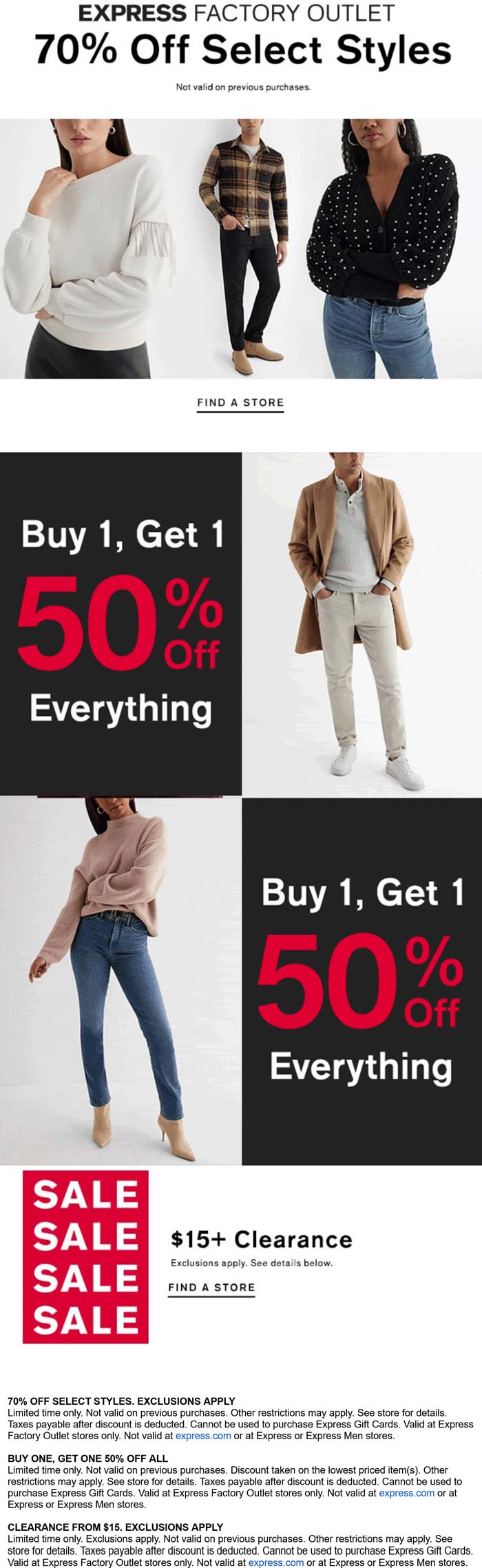**Express Factory Outlet Clearance Sale Advertisement**

The top of the advertisement prominently displays the Express Factory Outlet logo alongside a vibrant announcement of "70% off select styles" written in bold. This offer is explicitly noted as not valid on previous purchases.

Prominently featured in the center is an image showcasing two women and a man. The woman on the left is dressed in a stylish white shirt, whereas the woman on the right sports a sleek black shirt paired with blue jeans. Between them stands a man with his hand casually placed in his pocket, wearing a fashionable flannel shirt.

Below this image, a call to action encourages customers to "Find a store," followed by another bold promotional text: "Buy one, get one, 50% off everything." This offer is visually impactful with "buy one, get one" in white text and "50% off" emphasized in larger, red font, repeated again in the lower right section of the advertisement.

In the upper right, another image features a man in a chic brown coat with his hands in the coat pockets. He is also seen wearing white shoes, white pants, and a dress shirt, highlighting a sophisticated ensemble.

On the bottom left of the advertisement, a woman is shown wearing a loose, larger cut shirt, paired with blue jeans and high heels. Below her, a red box is marked with multiple mentions of the word "SALE" and highlights "$15 plus clearance" items. It also notes that exclusions apply, directing viewers to see the detailed terms below.

The footer of the advertisement is filled with three paragraphs of detailed terms and conditions, ensuring customers are fully informed about the sale's specifics.